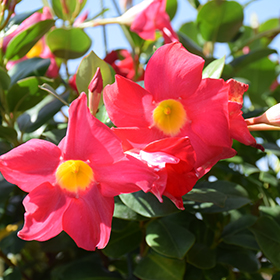This image is a square photograph prominently featuring two large, bright pink hibiscus flowers with striking yellow stamens and pollen at their centers. The blossoms, with approximately five petals each, radiate from the circular yellow centers and are wide open, capturing immediate attention in the foreground of the shot. Surrounding these primary pink flowers are lush green, oval-shaped leaves forming a backdrop that fills most of the picture. In the background, other flower buds can be seen, though none are as prominent as the two main hibiscus blossoms. The sky above the greenery is a clear, light blue, indicating a sunny, cloudless day - possibly around noon - as evidenced by the shadows cast on the flowers. The combination of the vibrant pink petals, green leaves, and blue sky creates a vivid, cheerful scene reminiscent of a tropical locale like Hawaii.